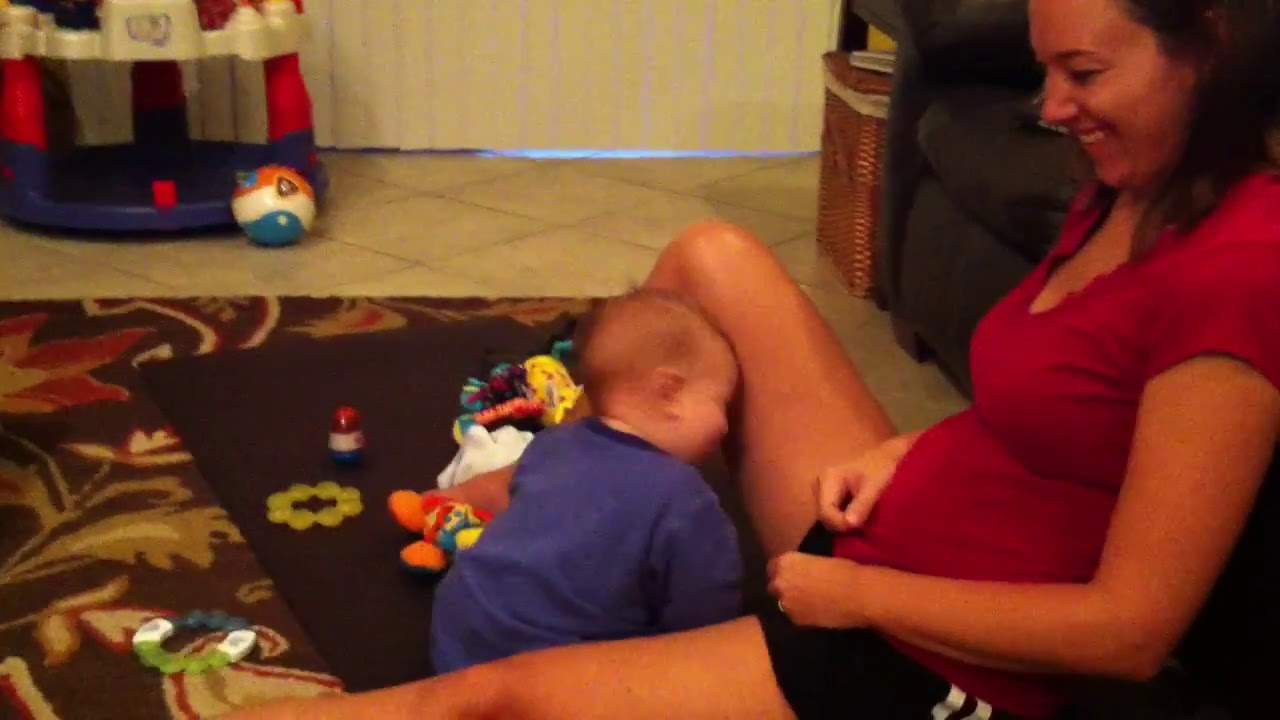A woman, positioned on the right side of the image and leaning on a brown couch, gazes down and laughs at a baby nestled between her splayed legs. She is dressed in a red short-sleeve t-shirt and black shorts with white stripes. The baby, donning a blue onesie, pushes its head against one of her legs while seated on a decorative rug featuring green and orange floral patterns. Atop the rug is a brown t-shirt play mat scattered with various baby toys, including a yellow circle-shaped teething toy and a white stuffed animal. In the background, a baby walker is visible along with a set of blinds, a tile floor, and a basket beneath an end table.